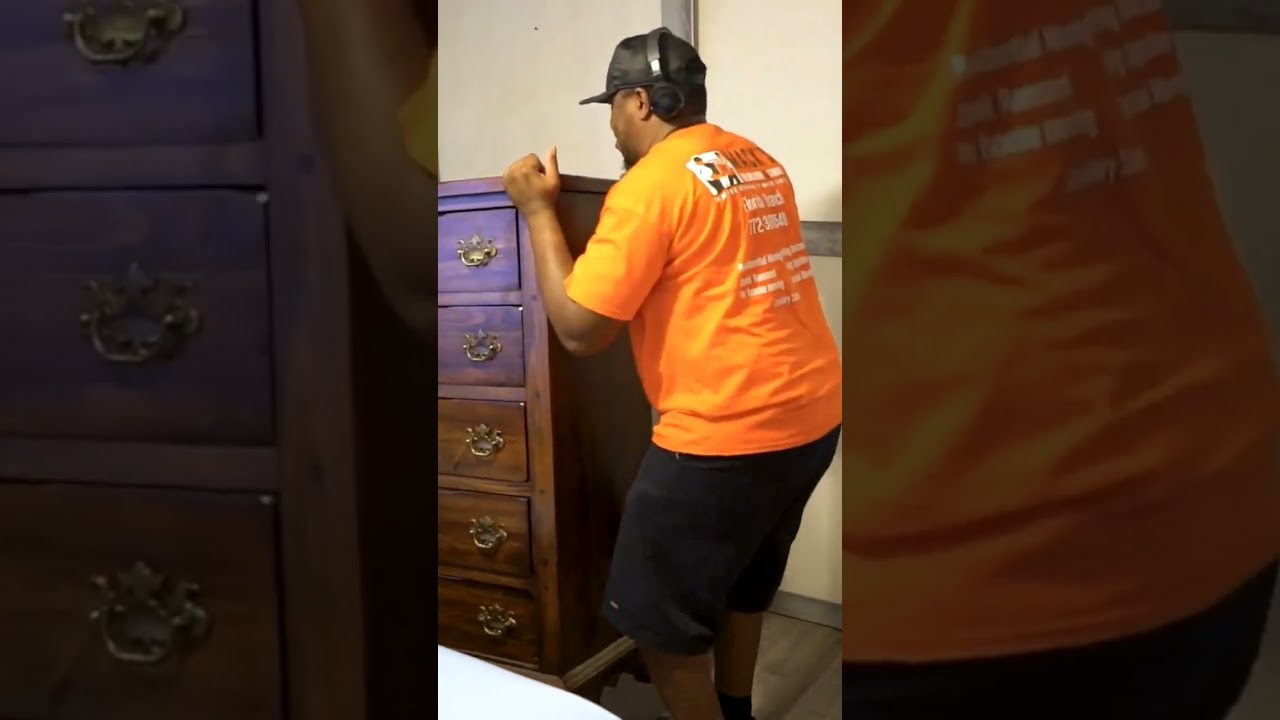In the image, an African-American man, likely a mover, is central as he attempts to lift a large, wooden chest of drawers with gold handles. He is wearing an orange work shirt featuring white text related to a moving company, black shorts, black socks pulled up high, a black ball cap, and black headphones positioned behind his ears. The man is slightly bent at the knees, ready to lift the chest, which is positioned to his left. The background includes a cream-colored wall with a hint of gray and a bed with white sheets visible in the foreground near his left knee. The image is detailed with focus on both the man and the dresser, showing a typical day in the life of a mover.